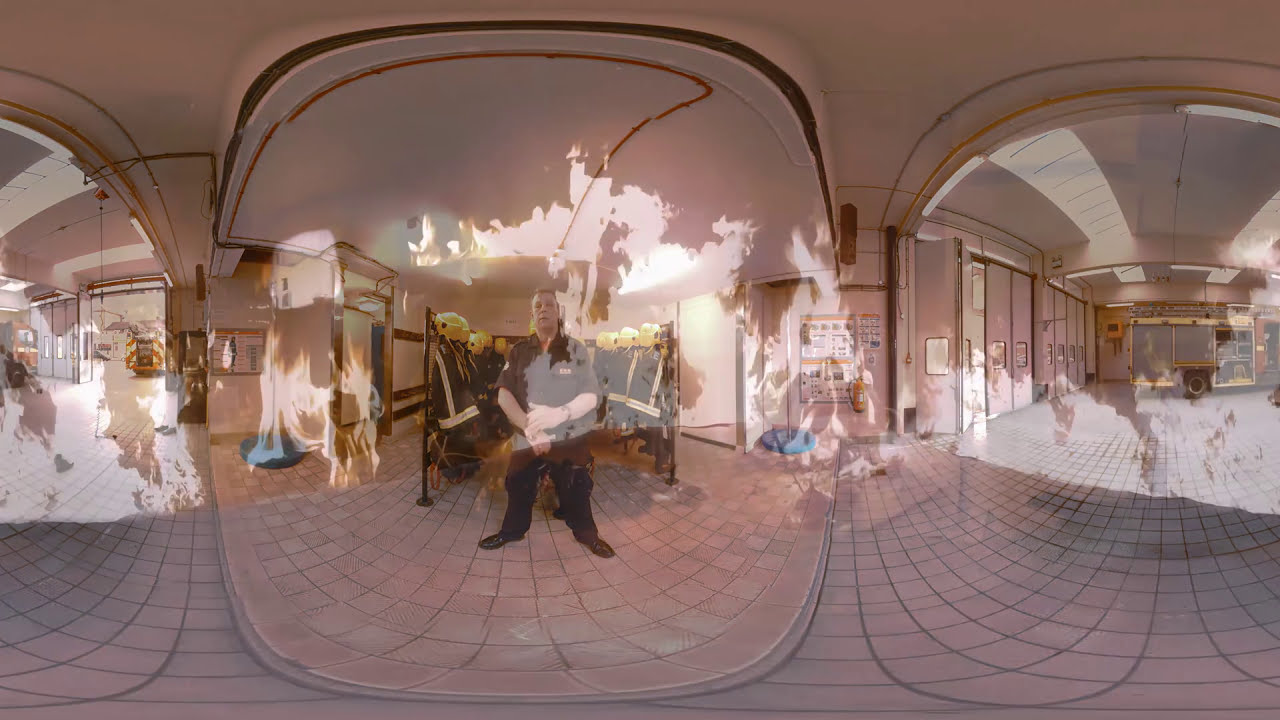This panoramic, 360-degree image presents a detailed, immersive view of a firefighter's station, segmenting into three distinct parts but forming a comprehensive scene. The central figure is a man, clad in a black short-sleeved button-up shirt, black pants, and brown shoes, standing resolutely with his arms crossed. Behind him, rows of fireman uniforms, distinguished by their black fabric with white and yellow stripes and yellow helmets, affirm the impression that he is a firefighter. The floor, composed of upscale white tiles, contrasts with the beige walls, enhancing the tidy appearance of the station. An overlay of flames superimposed onto the image contributes a ghostly ambiance, creating the illusion that the room is engulfed in fire.

On the left side of the panoramic view, you can discern a garage-like door revealing a fire truck outside, further attesting to the setting being a firefighter's station. The right side continues the immersive experience with what appears to be pink, restaurant-style swinging doors, possibly leading to another area within the station. The overall scene intricately blends textures and realities, from the tidy, upscale interiors to the ethereal overlay of flames, making it both captivating and somewhat deceptive, reinforcing the multifaceted duties and environments firefighters navigate daily.